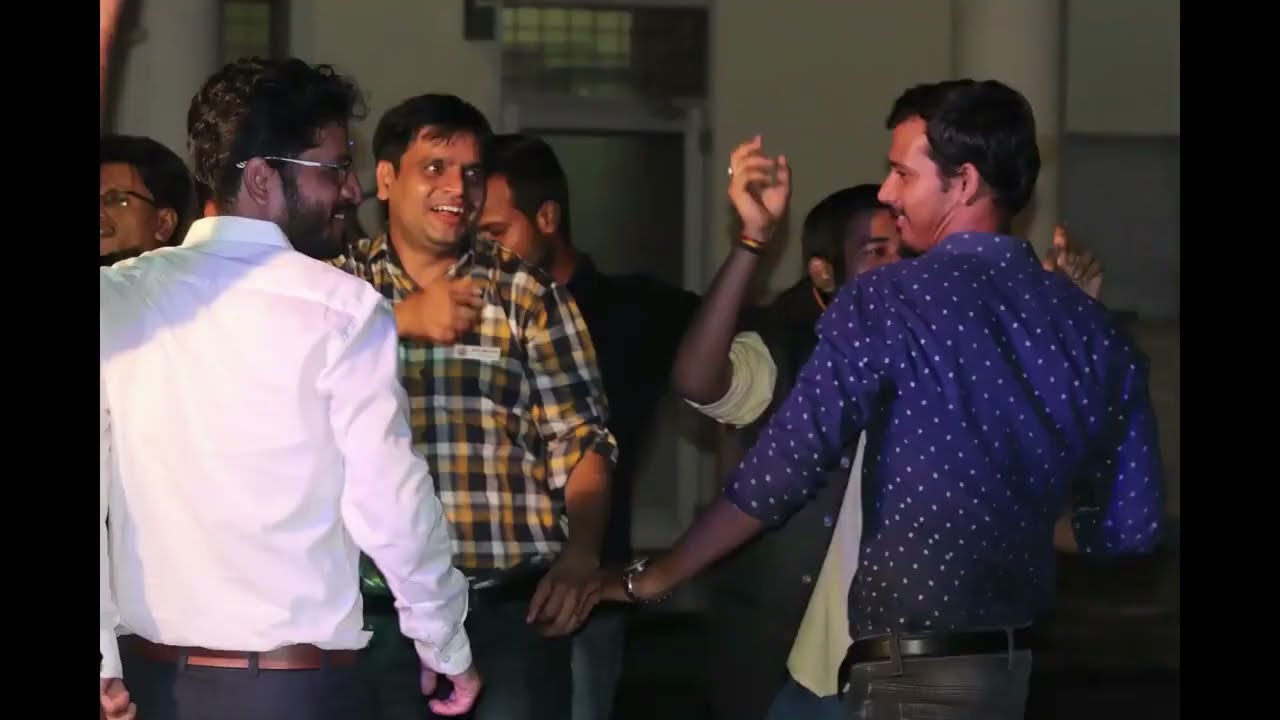The image shows a lively group of men, likely of South Asian descent, engaged in energetic dancing, possibly at a wedding or formal celebration. They all have light brown skin and black hair. On the left, a man with his back turned wears glasses, a white dress shirt, black dress pants, and a brown belt. In front of him, another man takes center stage, smiling with his mouth open and one hand lifted, dressed in a yellow flannel shirt and black pants. Towards the right, a man in a blue shirt with white dots and a watch is also in mid-dance, with his body partially turned to the side. In the background, additional dancers can be seen, contributing to the festive atmosphere. The room they are in has a white wall that appears yellowish due to warm lighting. A distinct feature in the background is a glass door with a white frame and an upper window displaying a grid pattern. The overall scene is one of joy and celebration, captured within a bordered photograph that emphasizes the formal attire of the participants, suggesting a significant event.